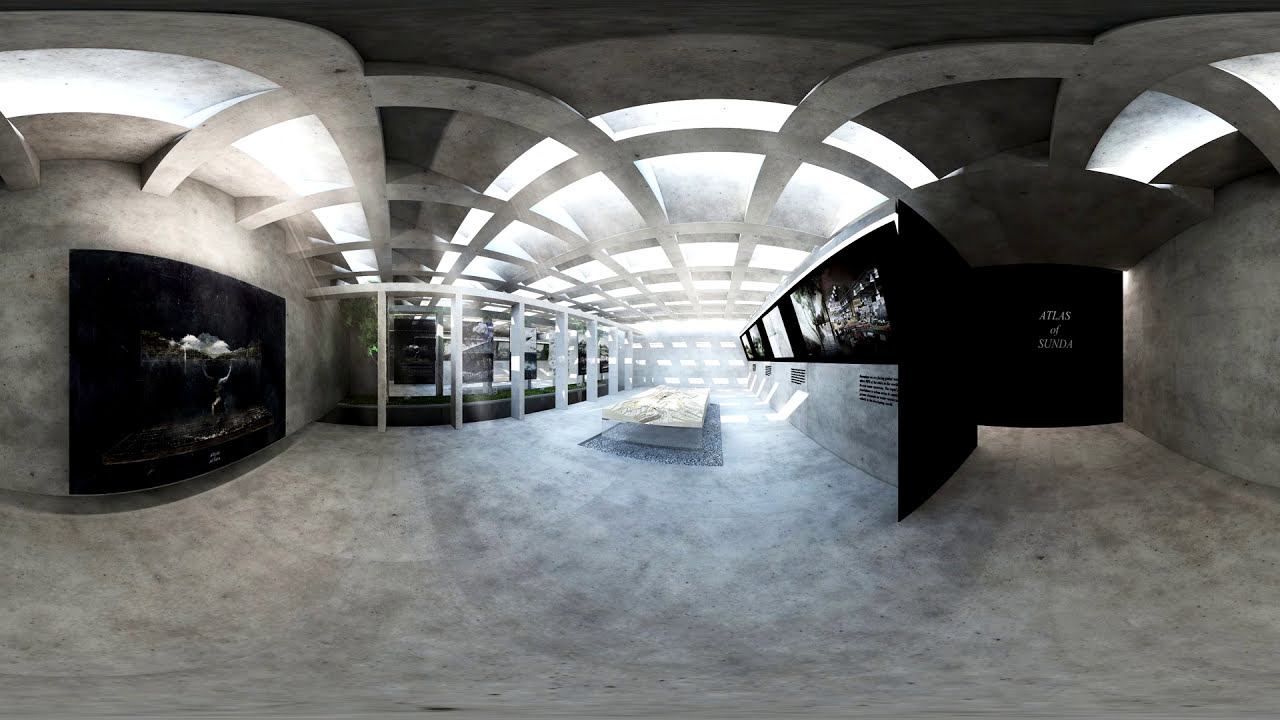The image depicts a highly luxurious, expansive indoor space dominated by white stone or marble textures on the floors, walls, and ceiling beams. The most central feature is a large stone granite table positioned prominently in the middle of the room. Surrounding the table is an open area with a grid-like structure allowing light to filter through, giving the room an airy, spacious feel. Off to the left, a sizeable aquarium adds a touch of vibrant green, contrasting with the otherwise monochromatic color scheme of gray, black, white, and some brown. Also on the left, there's a large screen, possibly a big-screen TV, contributing to the modern aesthetic. The right side of the room features an array of televisions or screens mounted on the wall, with several of them arranged in a linear formation, accompanied by some indistinct text beneath. One notable text visible towards the right side reads "Atlas of Sunda," suggesting a theme or focal point for the room. Overall, the room exudes opulence and modernity, with a balanced mix of natural stone elements and high-end electronic devices, set within what appears to be an extensive, warehouse-style building.